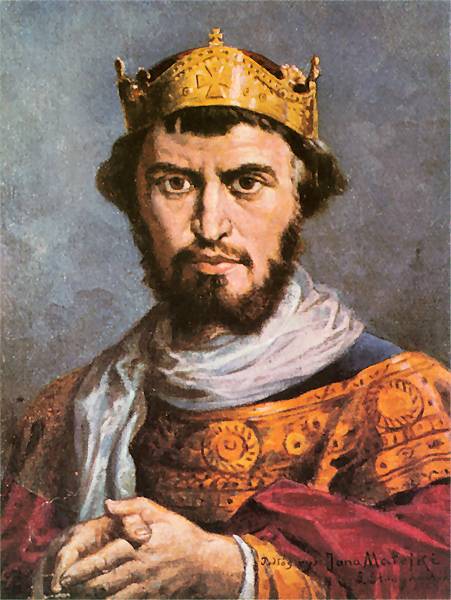This is a highly detailed painting of a regal-looking Caucasian man with a full beard and brown hair, appearing to be in his 50s. He is adorned in an elaborate outfit featuring shades of red, gold, orange, and a blue shirt beneath. A white scarf is wrapped around his neck, adding to his majestic appearance. His dark brown eyes convey a stern expression. Atop his head, he wears a gold crown with a cross symbol. The man’s hands are clasped together in front of him, clearly visible. The backdrop is a varying shade of gray, emphasizing the subject without any additional objects or text in the image. The central composition of the portrait further highlights the man as the sole focus, suggesting an aura of authority, possibly depicting a king or nobleman from the 15th or 16th century. The painting is signed, but the signature is illegible.